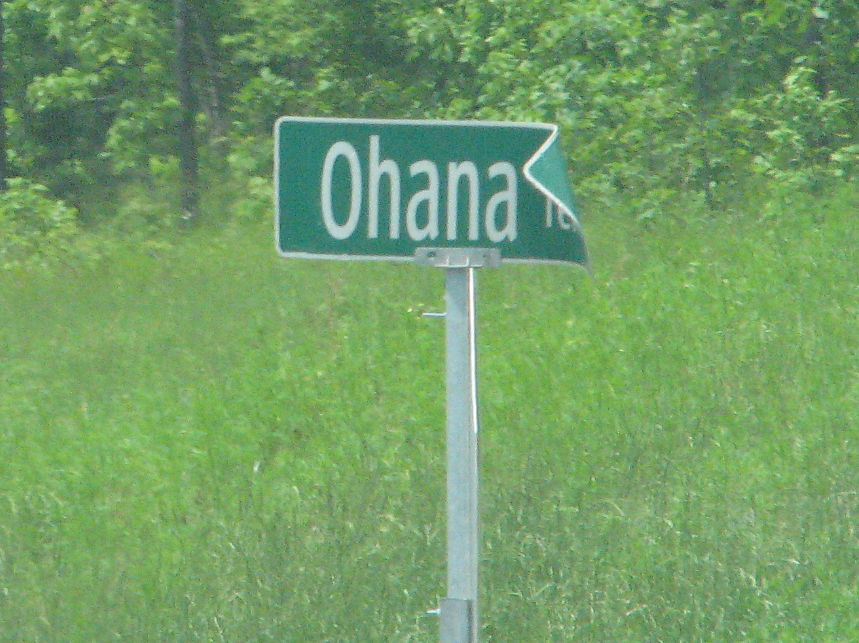This photograph features a slightly bent green rectangular street sign. The sign, which is affixed to a metal pole, displays the word "Ohana" in white letters, though part of the sign is obscured by a curve, making it difficult to distinguish the full text. The pole appears firmly planted in the ground. Surrounding the sign is a lush, verdant backdrop filled with tall grasses, bushes, and a dense wall of trees, showcasing a variety of greens and browns that contribute to the natural beauty of the scene.